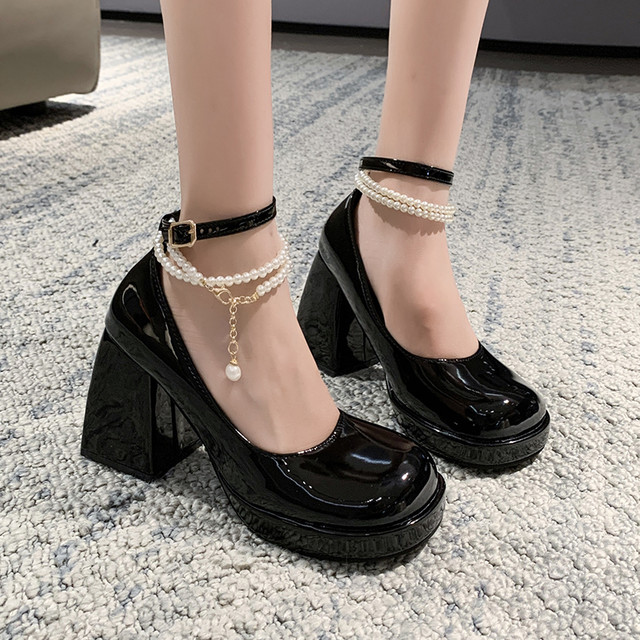In the image, you see a close-up of a Caucasian woman's feet adorned in striking, black shiny vinyl boots that have a cartoonishly exaggerated design. The boots feature substantial platform bottoms and thick, square block heels. Thin black straps with gold buckles secure the boots around each ankle. Around each ankle, you also notice double-layered pearl anklets with a gold clasp and a dangling gold chain with a larger pearl at the end. The woman, who appears to be modeling the boots, is standing on a highly textured gray carpet with darker lines running through it. In the background, you can make out the bottoms of light brown furniture, possibly a couch or chair, although the image remains focused on the footwear and does not provide much detail about the surroundings.